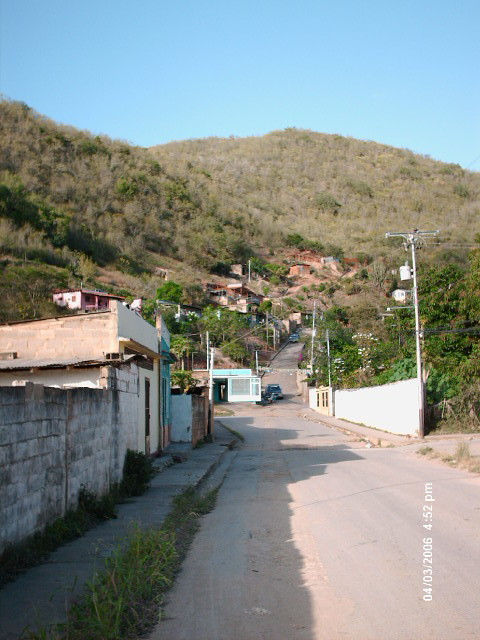The photograph captures a rural scene dominated by a lush green hill. The hill, covered in various shades of greenery including grasses, bushes, and a few trees with brown trunks, extends across the top and center of the image. At the base of the hill, a small street runs diagonally from the bottom right to the upper area, bordered by concrete walls and shadow-casting buildings. The street itself appears grayish-white, flanked by sidewalks with sporadic patches of grass. The left side of the street is lined with various single-storey buildings, some looking ramshackle and possibly indicative of a lower-income area. These buildings include white, blue, and pink structures, with flat roofs and garages, interspersed with white light or telephone posts. Cars are parked along the road, though their details are indistinct due to distance. A distinctive white wall also runs along the right side of the street. Above all, the sky is a clear light blue, adding a serene backdrop to the somewhat dilapidated foreground. Overlaid on the bottom right corner of the image in white text are the date "04-03-2006" and the time "4:52 PM," tilted slightly to the left.